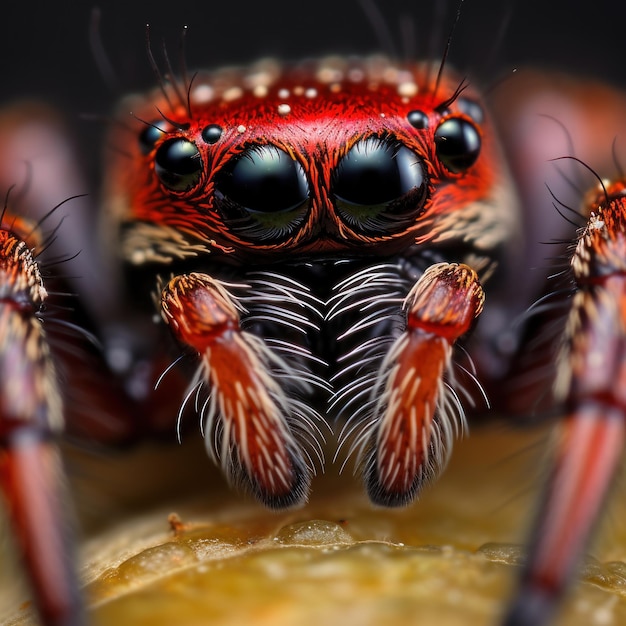The image shows a highly detailed close-up of a tarantula, captured with sophisticated microscope equipment. The tarantula features two prominent black eyes at its center, flanked by two smaller eyes on either side, and two additional eyes slightly above them. Its face is adorned with small, beady fangs, and the body and legs are covered in an abundance of fine hairs. These hairs are primarily white along the sides and near the body, with darker, almost black hairs mixed in at the tips of the legs. The legs themselves exhibit a dark red coloration. The tarantula's back features small, white, rock-like spots, possibly serving as camouflage. The image captures the spider's intricate details so clearly that it almost appears to be a photorealistic drawing.